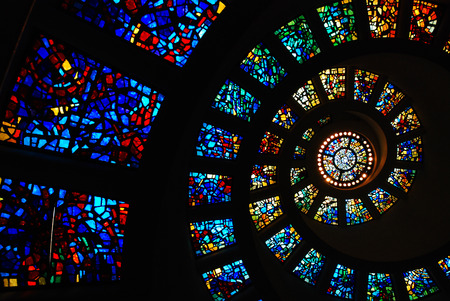This photograph captures an intricate arrangement of stained glass panels forming a mesmerizing spiral pattern that ascends upwards, culminating in a circular stained glass window. The rectangular stained glass panels, framed by black dividers, are meticulously spaced and feature an array of vivid colors including cobalt blue, aqua blue, red, golden yellow, pale yellow, orange, and white. These individual panels do not depict specific images but serve as decorative elements, contributing to the overall aesthetic with their vibrant hues. The stained glass windows spiral inward, with the largest panels appearing on the left side, likely due to their proximity to the viewer. As the spiral narrows towards the center, the panels become progressively smaller, drawing the eye upwards to the circular window at the top, which is outlined by a string of white, round lights. This central circular window may be positioned at the apex of a dome, completing the captivating visual journey from the periphery to the heart of the design.